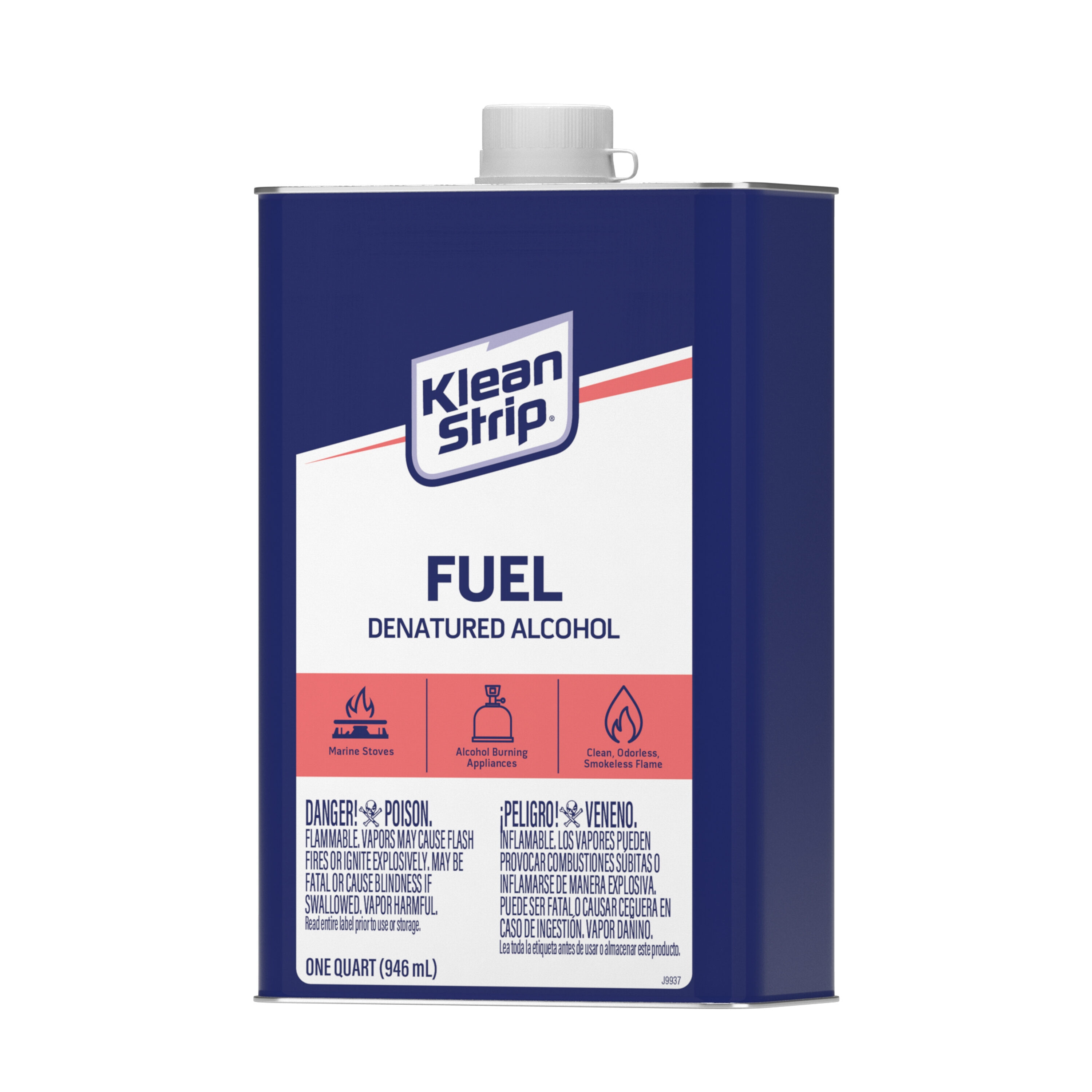The image depicts a blue, squared-off can labeled "Klean Strip" across a white background section with an orange stripe. The can features a white plastic cap with a thin silver lining at the top. The main text in blue reads "Fuel" with "Denatured Alcohol" underneath. The design includes three illustrations within the orange stripe: one with a flame icon that says "Marine Stoves," another with a small bottle labeled "Alcohol Burning Appliances," and a third flame icon stating "Clean, Odorless, Smokeless Flame." Below these illustrations are warning signs, including a skull and crossbones indicating poison, and various safety warnings in both English and another language. The bottom left corner of the can specifies the volume as "One Quart, 946 milliliters."